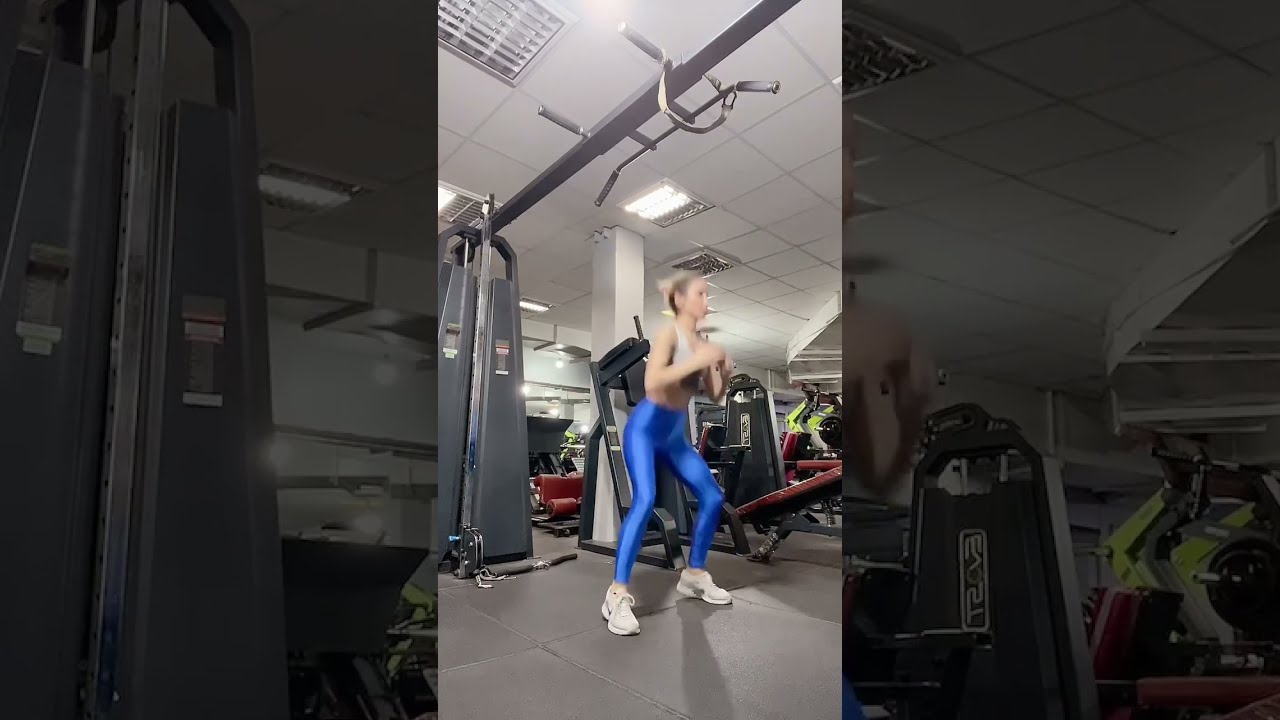The image features a white woman exercising in a well-lit gym with a white drop ceiling. She is front and center of the composition, performing a squat with her hands clasped together and her knees bent. She is clad in a white sports bra and strikingly bright, neon blue, form-fitting leggings, complemented by white sneakers. Her blonde hair is tied back tightly. Surrounding her, various gym equipment is visible: on her left, a black machine with pulleys and to her right, several machines with red pads designed for seated workouts. The gym also features a rocky concrete floor, vents in the ceiling, and some ceiling lights, adding to the well-lit yet slightly dim ambiance. The image is flanked on both sides by darkened, zoomed-in panels of the main scene, emphasizing the gym equipment visible in the central frame. The entire setting captures the dynamic energy of a gym environment.